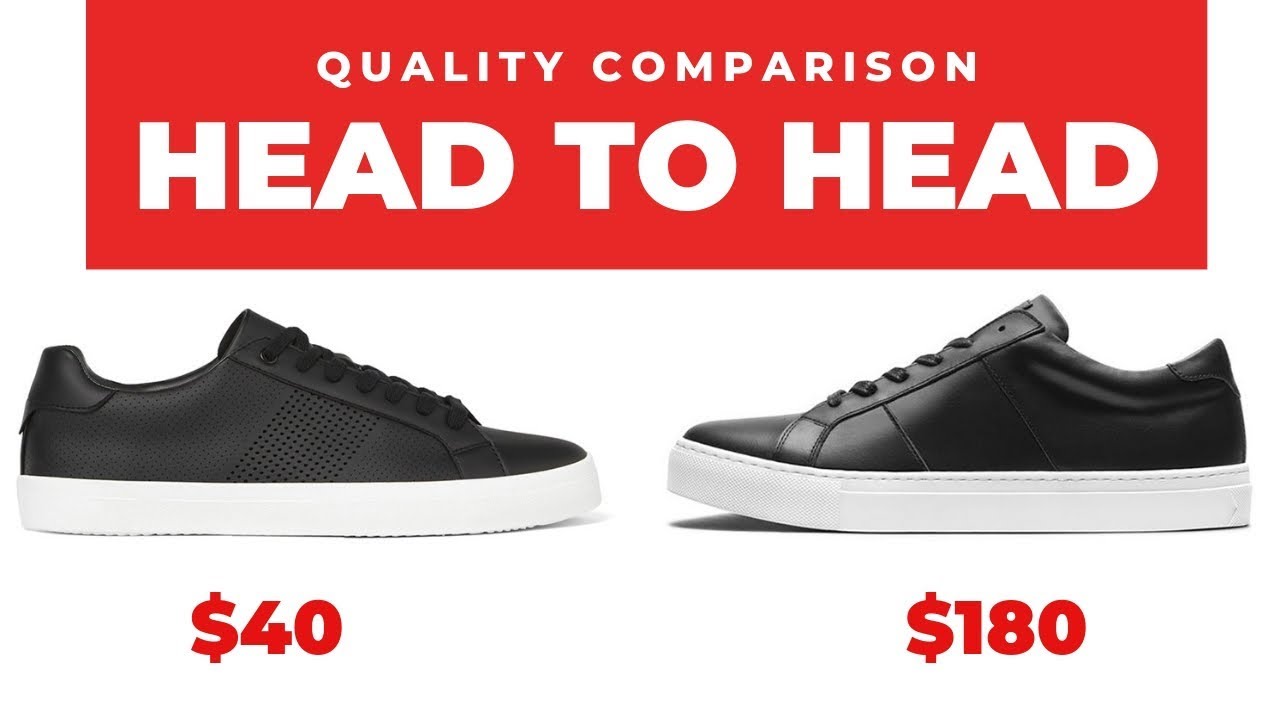The image is an advertisement titled "Quality Comparison Head-to-Head" displayed on a bold red rectangular background with white stencil-like text. It features two black athletic sneakers with white rubber soles facing each other. On the left, the sneaker, which is priced at $40, appears to have a cloth or canvas upper with a pattern or holes, indicating a lower quality. In contrast, the sneaker on the right, priced at $180, has a sleek and smooth leather upper, suggesting higher quality and sophistication. Both sneakers are similar in color scheme but differ notably in material and presumed durability. The background of the image is white, and the contrasting price points are prominently highlighted in red beneath each respective shoe. The ad effectively compares a high-end $180 sneaker to a more affordable $40 option, showcasing their similarities and differences in design and quality.